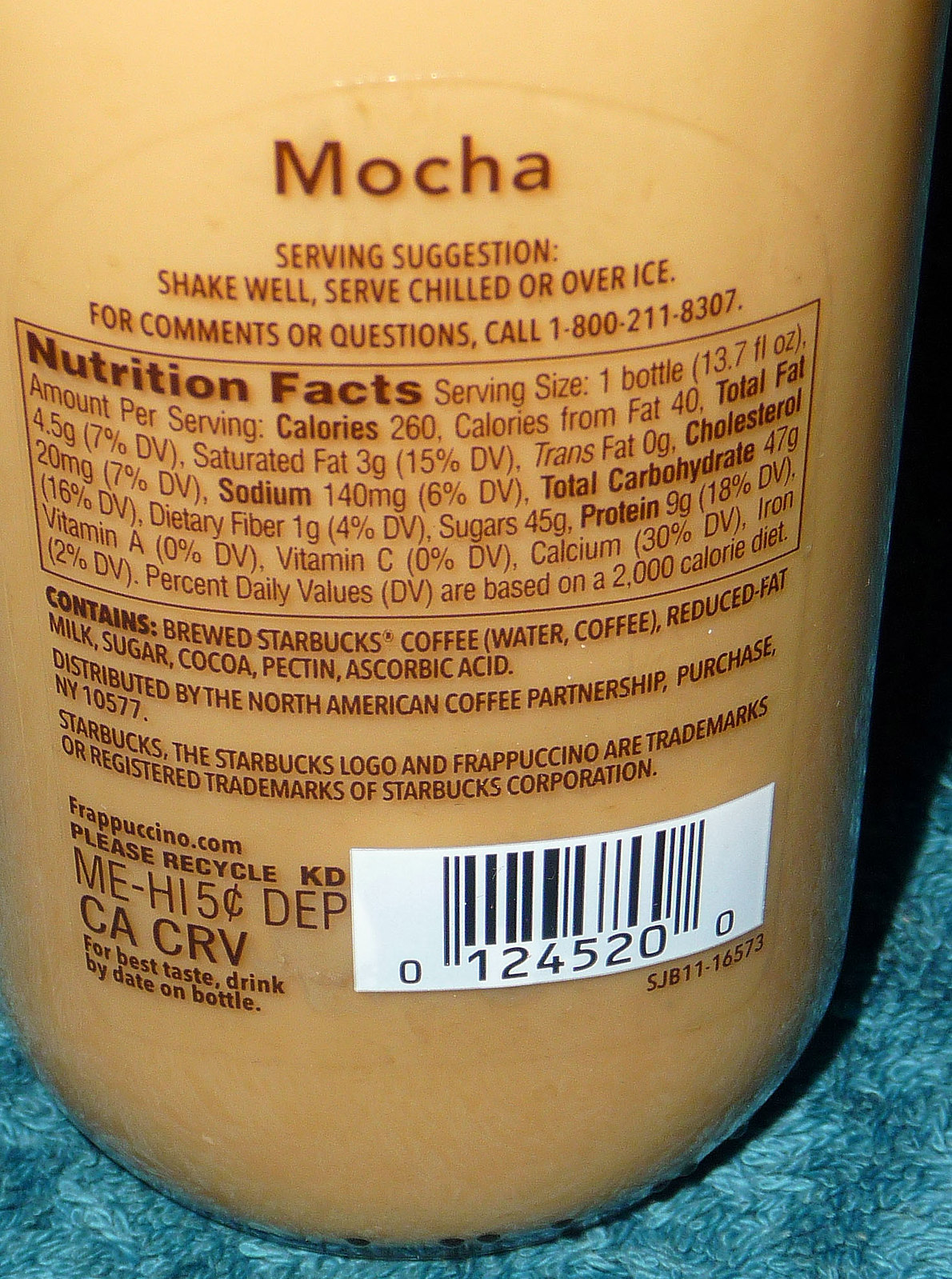The image captures a close-up of the back of a Starbucks mocha Frappuccino coffee bottle, set against an aquamarine towel with a terrycloth texture. The vibrant background enhances the clear bottle, inside which the creamy coffee beverage is visible. The label at the top clearly reads "Mocha," followed by serving suggestions: "Shake well, serve chilled or over ice." The label also provides a contact number for comments or questions: 1-800-211-8307. The nutrition facts state a serving size of one 13.7-fluid-ounce bottle, containing 260 calories and 4.5 grams of total fat (7% of daily value), including 3 grams of saturated fat (15% of daily value). The ingredients listed include brewed Starbucks coffee, reduced-fat milk, sugar, cocoa pectin, and ascorbic acid. Additional information on the label includes recycling instructions, deposit details for Maine and Hawaii, the California CRV, and a UPC code on a white label with black lettering. The product is distributed by the North American Coffee Partnership and carries the trademarks of the Starbucks Corporation.